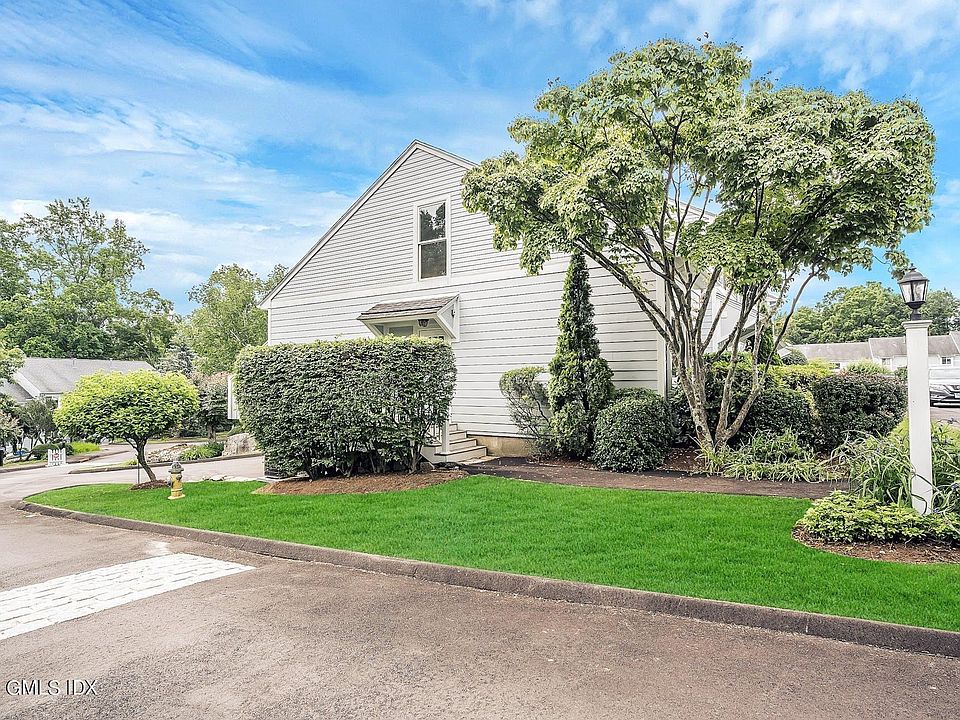This detailed image showcases the exterior of a white house shot from the side, emphasizing the well-manicured lawn adorned with neatly trimmed bushes and trees. The bright green front lawn adds vibrancy to the scene, set against a backdrop of a blue sky with some clouds. A white light post stands prominently next to a walkway leading to white wooden steps that ascend to a door partially obscured by shrubs. A single window is visible above the door, adding architectural interest. On the right side, a smaller tree and a peculiar yellow fire hydrant are situated near a curb on the grass, which borders what appears to be a driveway or street area. In the left background, another house, partially obscured by a tree, can be seen. The colors and lighting have a slightly artificial quality, suggesting the image might be augmented reality-generated, with an odd contrast between the bright sky and the seemingly cloudy illumination of other elements. The photograph also features white text at the bottom left corner reading "GMLS IDX." This horizontal image captures both the charm of the house's landscape and the slightly surreal ambiance of the scene.